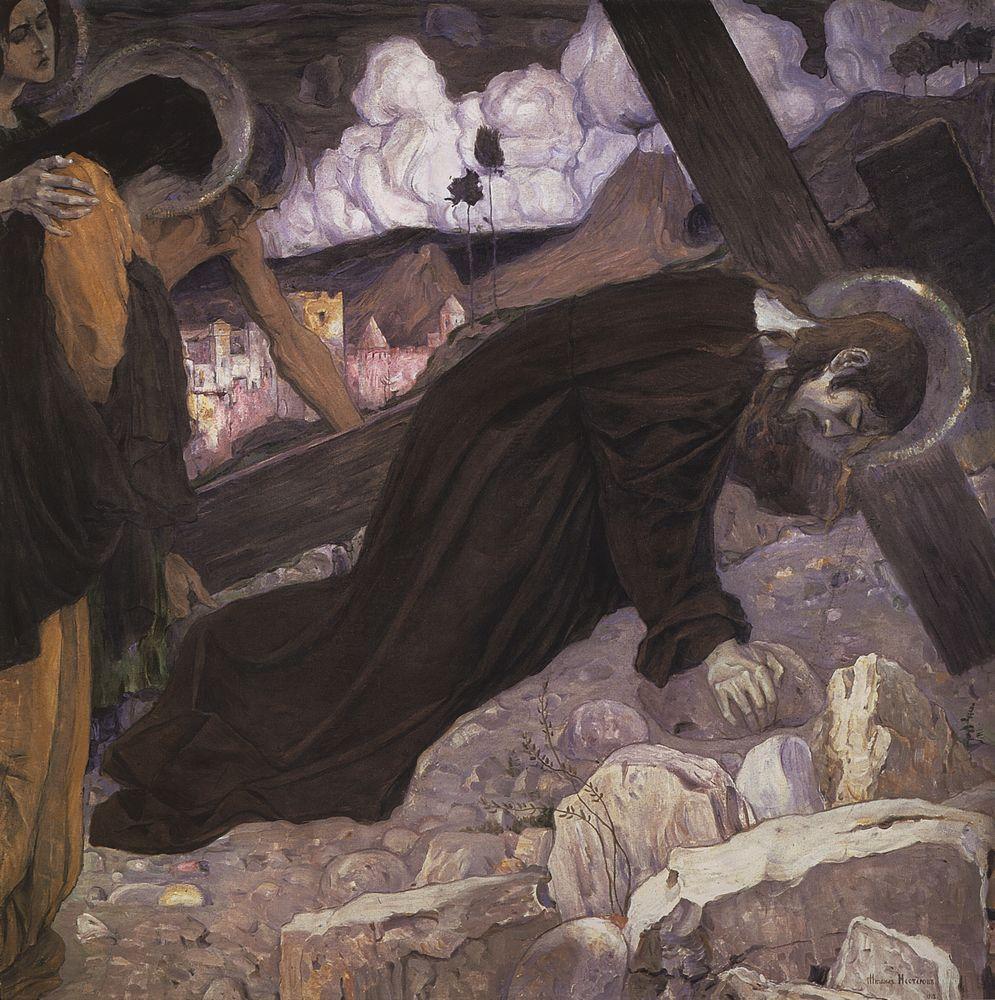In the painting, the central figure, likely Jesus Christ, is depicted kneeling on the ground, wearing a brown robe. His long brown hair falls forward as he appears to be staring at the ground, with his eyes closed, next to a wooden pillar that seems reminiscent of a crucifix. His right shoulder bears a large cross, suggesting he is in the process of carrying it. A significant element is a golden halo around his head, indicating his sanctity. To the left of Jesus, there are other figures; one is a woman with a sad expression, reaching out a comforting hand towards another person who is bowed down with their hands over their face and also has a halo above their head. The background features a distant town with outlines of buildings, set against rolling white clouds and a dark, gloomy landscape dominated by various shades of brown and gray. The overall tone is somber, with strong religious connotations, capturing a moment of struggle and compassion amidst a bleak, rocky hillside.